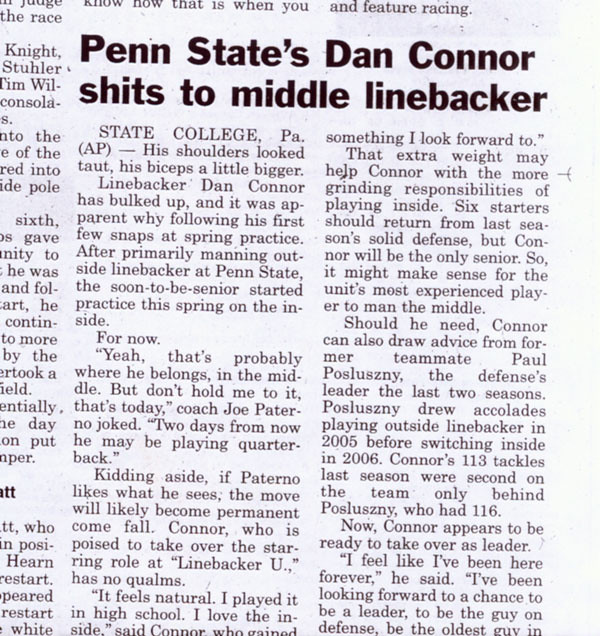The image depicts a scanned section of a newspaper featuring a clean, white background with black text, indicating a digitally preserved state. Dominating the scene is an eye-catching headline: "Penn State's Dan Conner Shifts to Middle Linebacker." The article, originating from State College, PA, via the Associated Press (AP), spotlights the physical transformation and positional change of Penn State linebacker Dan Conner. His shoulders appear taut, and his biceps seem larger, indicative of his bulking up. This physical evolution was evident during his initial snaps at spring practice. Previously an outside linebacker, the soon-to-be senior has commenced training on the inside this spring. A quote from Coach Joe Paterno humorously mentions that while Conner seems suited for the middle now, his position may still shift, perhaps even to quarterback. Conner himself, poised to take on a leading role at linebacker, expresses confidence and comfort with the change, recalling his experience playing the position in high school. The narrative details his journey and preparation for the upcoming role at Penn State.